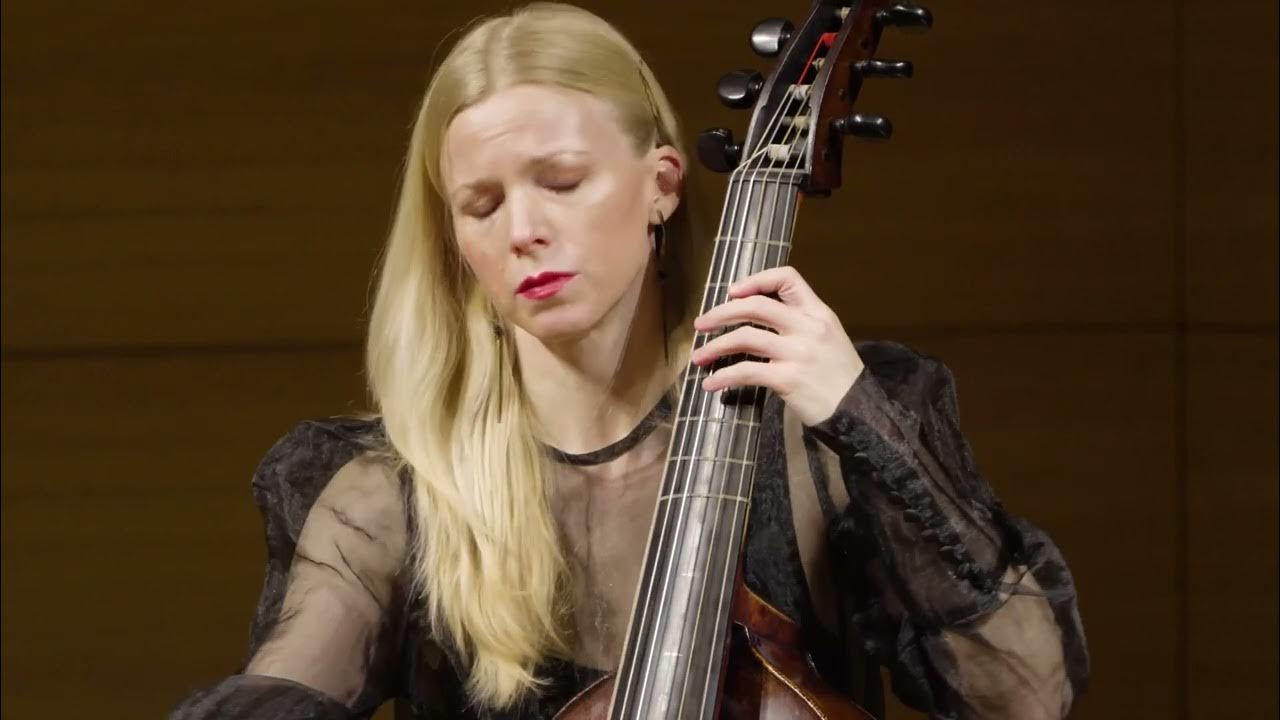In this captivating close-up image, a female musician with long blonde hair, styled with a middle part and swept to her right, is engrossed in her performance on stage. She is playing what appears to be a six-string upright bass guitar. Dressed in a sheer black long-sleeve top with a black tank top underneath, she exudes a powerful presence. Her eyes are closed, and her red lipstick stands out prominently against her fair complexion, capturing her deep focus and immersion in the music. Her left hand is placed on the fretboard, showing four fingers and a thumb, while her right hand is out of the frame. She is adorned with black hoop earrings and has furrowed eyebrows, indicative of her concentration on the melody she is creating. The background features a basic stage setup with dim lighting and wood panels, emphasizing the spotlight on her emotional and skilled performance.